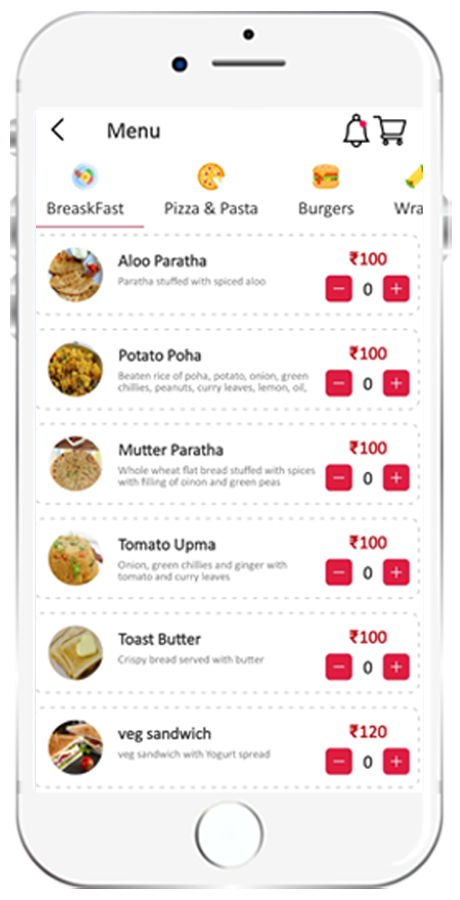The image showcases an old-style silver iPhone with a home button at the bottom. The device features three buttons on the left side and one on the right. At the top, there is a front camera and a prominent bar typical of older phone models. The screen displays a menu interface with the word "Menu" written at the top alongside a left-pointing arrow, a red notification bell icon, and a shopping cart icon.

Below the header, there are menu categories labeled "Breakfast, Pizza and Pasta, Burgers, and Wraps." Following the categories, there is a list of six items with their respective prices in an unknown currency: 

1. Aloo Paratha - 100
2. Potato Poha - 100
3. Mutter Paratha - 100
4. Tomato Oompa - 100
5. Toast Butter - 100
6. Veg Sandwich - 120

Each item has red plus and minus icons next to it, indicating quantity selections, all currently set to zero.